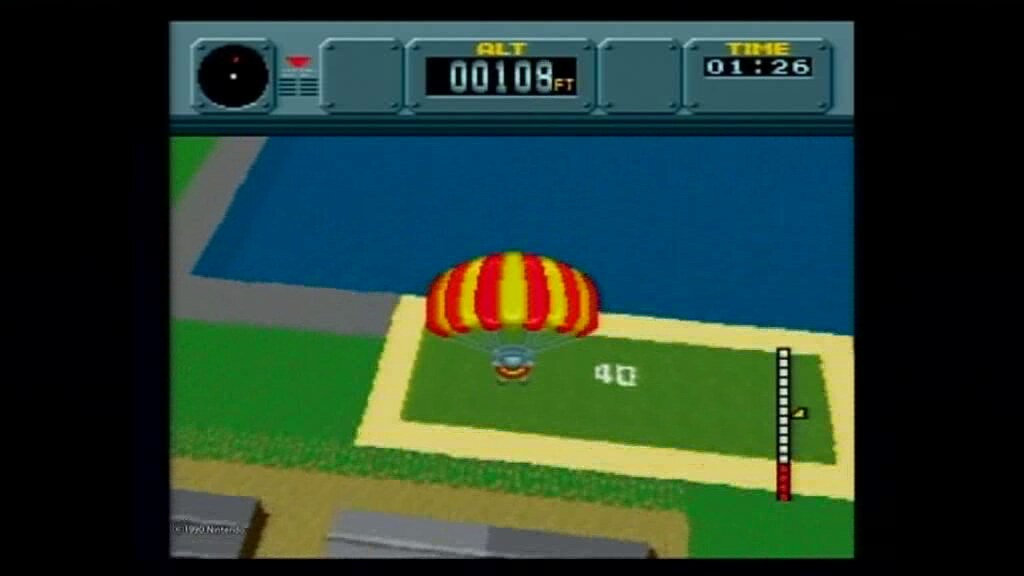The screenshot from the video game features a detailed, immersive in-game scene. At the top of the screen, a grayish-green bar displays critical information, including a timer set at 1 minute and 26 seconds, and an altitude reading of 108 feet. Below this bar is a rectangular section with a blue background and a gray border, followed by another rectangular shape with a yellow-green border, all set against a grassy area leading into a brown terrain with two gray segments.

In the center of the image, a character is seen parachuting down with a vibrant yellow and red striped parachute. The parachute's ropes extend down to a figure that appears to be floating away from the viewer. On the lower right side of the screen, there is a progress bar, adding to the gameplay dynamics. The overall color scheme and elements, like the light blue-gray backgrounds and the various bordered sections, enrich the visual complexity of the game environment.